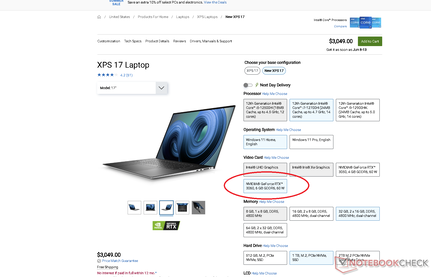**Caption:**

This image appears to be a screenshot of a website displaying an advertisement for a high-end laptop, specifically the XPS 17. The design layout includes various elements like menus and text bars positioned at the top. On the left side, the price of the laptop is listed as $3,049, positioned above a green "Add to Cart" button. The product name "XPS 17 laptop" is clearly visible, along with a star rating which seems to be either 4.2 or 4.3 stars, although the exact number is obscured due to blurriness.

The main image showcases the laptop featuring a blue and green screensaver and a grey keyboard. Below this main image are five smaller thumbnails, with the center thumbnail being selected. To the right, there is a "Choose your configuration" section, although the specific options are unreadable due to the small and blurry text. 

Highlighted configurations indicate that the middle processor option, Windows 11 Home English operating system, and the fourth video card option have been selected. Additionally, the third memory option and the second hard drive option are chosen. These selections are further marked by various indicators, such as grey buttons and a red oval that is superimposed over the image, particularly around the chosen video card.

The lower right corner of the screenshot features a small watermark with the outline of a laptop. Accompanied by the text "notebook" in red, it includes partially visible letters "C-H-E-E-C" and an almost certain "K," written in a greyish-black color.

Overall, the image captures the detailed layout of a product listing page, highlighting the various customizable options available for the XPS 17 laptop amidst a somewhat blurred interface.